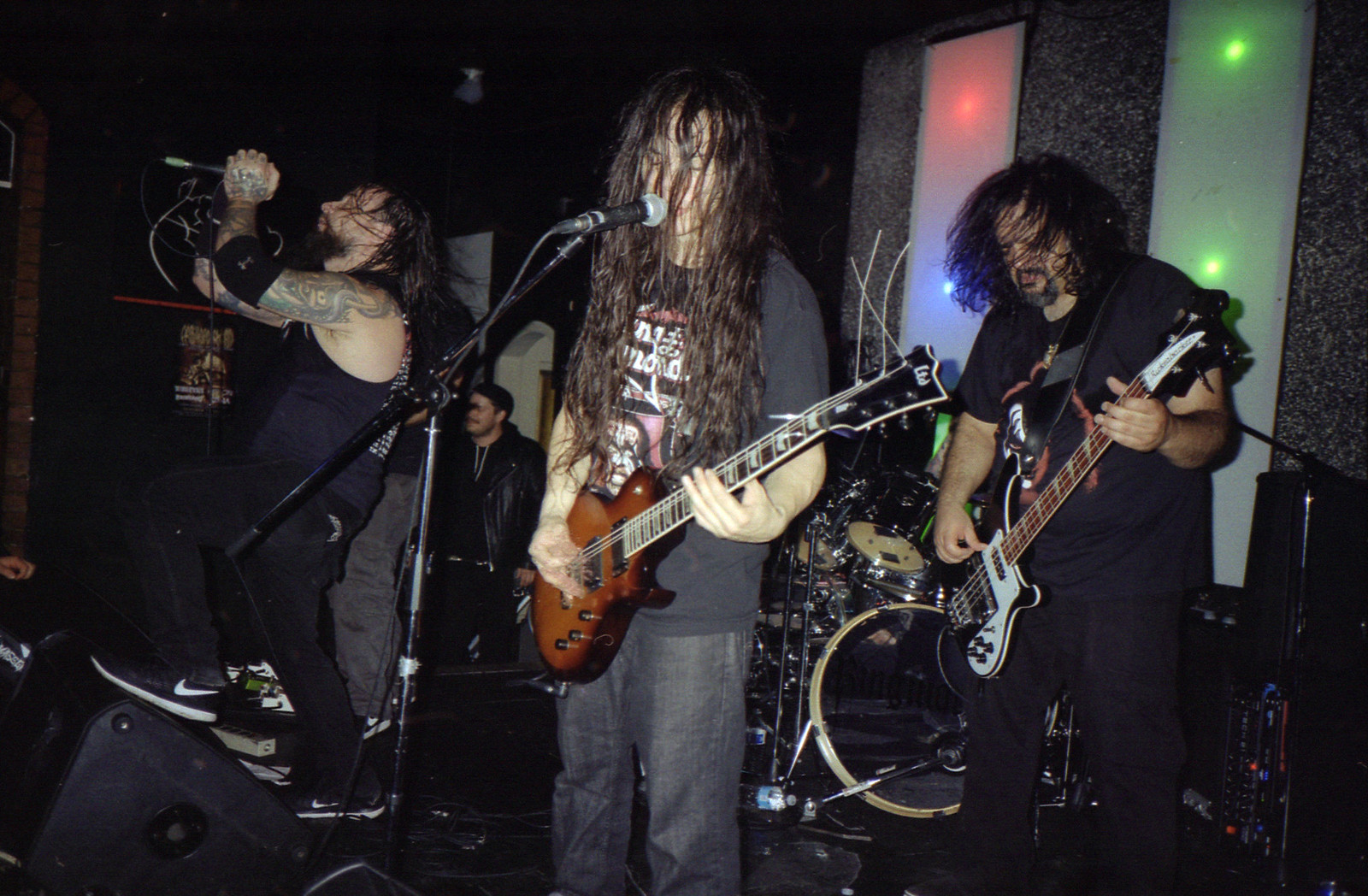The photograph depicts a live performance by a grunge rock band on a small, black-colored indoor stage. The lead singer stands at the forefront, gripping a microphone and wearing a sleeveless black tank top, black pants, and black shoes with white bottoms. His tattoos are visible on his arms, and his sweaty, stringy hair falls over his face. There's also an elbow wrap on one arm, adding to his rugged look. To his side, a guitarist with long black hair, clad in a black shirt and pants, plays a white and black guitar. Another band member with long brown hair, a black shirt, and gray jeans plays a brown bass guitar or another guitar. A drummer is positioned behind the musicians, partially obscured but identifiable by the metal drum kit. The stage setup includes large speakers, amplifiers, and various lights that cast green, red, and blue hues onto a gray backdrop, along with two windows that blend into the background due to the lighting. Additionally, a member wearing a leather jacket can be seen on stage. The overall atmosphere is gritty and raw, characteristic of a grunge band, with elements like a sprinkler head on the black ceiling adding to the intimate venue's detail.